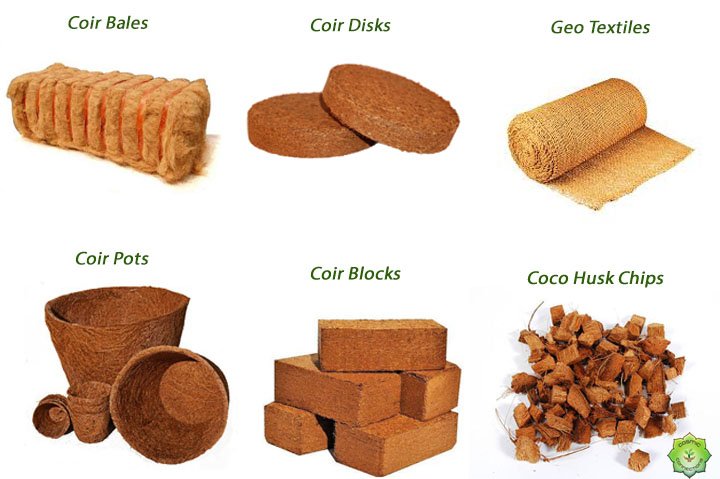The image showcases six types of natural, fibrous, hand-made items, each with a corresponding label. In the top left corner, there's a rectangular bale marked "Coir Bales (C-O-I-R B-A-L-E-S)," appearing as tightly packed bundles of brown fibers. Adjacent to this, labeled "Coir Discs (C-O-I-R-D-I-S-K-S)," are two stacked brown discs made of a fibrous material. To the right, under the heading "Geotextiles," is a roll of brown woven fabric, suggesting a versatile, spreadable fiber textile. In the bottom left corner, labeled "Coir Pots (C-O-I-R P-O-T-S)," there's an array of hand-woven brown pots, possibly biodegradable and suitable for planting. Centered at the bottom, "Coir Blocks (C-O-I-R B-L-O-X)" are depicted as brick-like shapes made from the same fibrous material. Finally, in the bottom right corner, labeled "Cocoa Husk Chips," we see a pile of dark brown chips, certified green compost, resembling wood chips used for gardening or mulching.